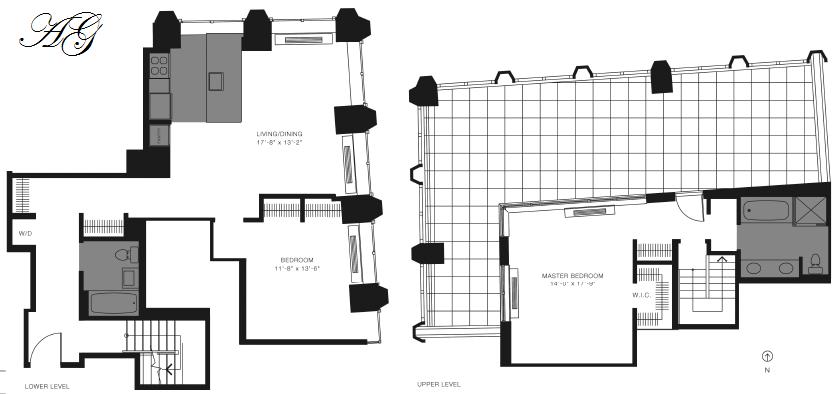This detailed blueprint depicts a two-story house design, with the lower level illustrated on the left side and the upper level on the right. In the upper left corner of the plan, "AG" is elegantly shown in cursive. The bottom left corner features a circular compass rose indicating the northern direction.

Starting with the upper level on the right side of the blueprint, there is an expansive deck or patio that extends leftward and wraps around the upper edge of the house. Three darker columns, likely support beams, are marked, along with lighter columns highlighted with black exteriors and white interiors, encircling the deck. Within the interior space of this level, beginning from the bottom left, the layout includes the patio followed by the master bedroom, which boasts a walk-in closet and potentially a fireplace (though it might also be a window overlooking the deck on the left and another window facing the top of the image). Exiting the bedroom involves a slight slant leading to another closet positioned behind the walk-in closet. Further along, there are stairs leading down to a landing and continuing downward. Heading directly forward from the stairs is a small ante room that leads into a bathroom equipped with a shower, bathtub, double sinks, and a toilet. There is also a door across from the stairs, opening onto the balcony/patio area.

On the lower level, starting from the right corner, an entryway leads into a hallway. Immediately to the right are stairs ascending to the upper level. Continuing down the hallway, there is a bathroom on the right side featuring a sink, toilet, and bathtub. Adjacent to the bathroom, on the left, are a washer and dryer cupboard and a linen closet. The hallway then turns to the right, with another closet situated on the right-hand side, adjacent to the bathroom. Proceeding straight ahead, the pathway opens into a combined living and dining area located in the back right corner. This space is defined by large black posts, presumably support beams. The kitchen occupies the upper left-hand side, accommodating a refrigerator, counters, and a stove. The living and dining room area is specified as 17.8 by 13.2 feet. In the bottom right corner, a doorway from the living room leads to a bedroom featuring a double closet, with the bedroom dimensions being 11.8 by 13.8 feet.

Overall, this house plan delineates a well-organized, two-story residence with thoughtfully allocated spaces for functional and leisurely living.